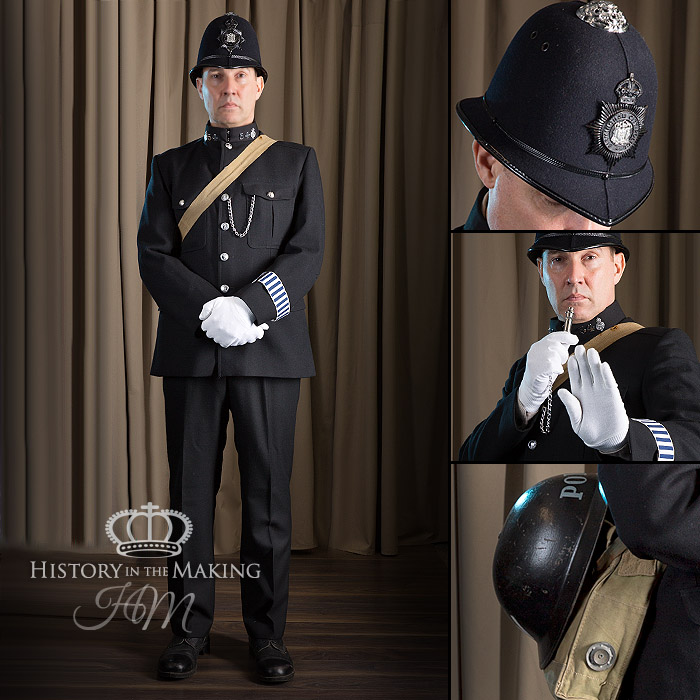The image is divided into two main segments: a large left section and a smaller right column. The left section, which occupies about two-thirds of the image, shows a full-length, professionally photographed portrait of a police officer dressed in an old-style, black British police uniform complete with white gloves. The officer stands on a dark wood floor against a taupe curtain backdrop, clasping his hands together and facing the camera. The uniform features distinctive details such as a shoulder band, a chain from his suit jacket, and a helmet adorned with a crest logo. At the bottom left of this section, overlaid with a crown illustration, the text reads "History in the Making, H.M."

The right column is divided into three equal-sized squares. The top square contains a close-up of the officer's helmet, clearly showing its crest. The middle square captures the officer with a whistle near his mouth, making a 'stop' gesture with his white-gloved hand. The bottom square depicts a close-up of a brown bag slung over the officer's shoulder, with the helmet attached to it.